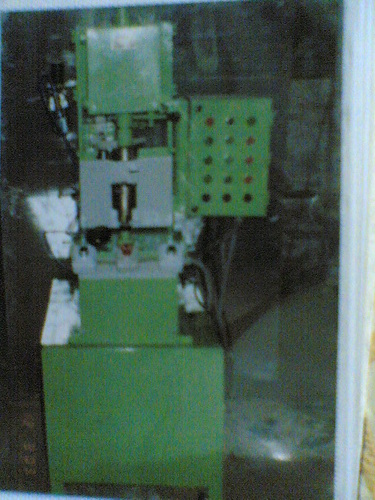The image shows an older, grainy photograph of a rather large, green-painted piece of machinery housed in a cramped room with a white doorway. The machine is primarily green with a few silver or grey metallic components. Central to the structure is a steel post or pole. On the right side of the machine, there is a separate box featuring a grid of buttons, arranged three by five. Additionally, there are some white cotton balls or similar objects stored in or near the machine's compartments. A grey plate with a gold tube runs through it, descending into the lower part of the machinery, though the exact function of this apparatus remains unclear.